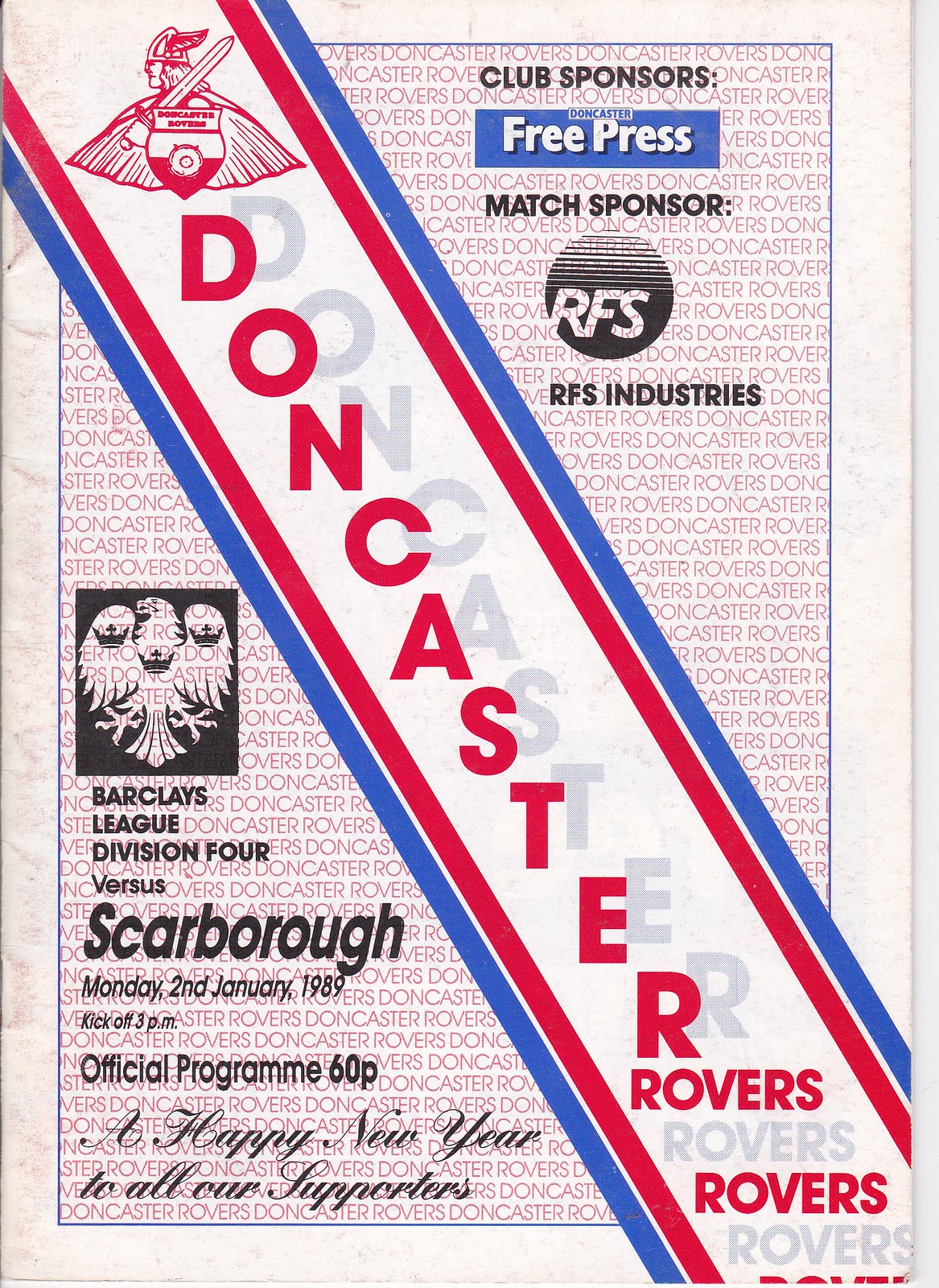This vertical rectangular image appears to be the front cover of an official program for a sporting event. The cover features a central diagonal white ribbon running from the upper left to the lower right, bordered by red lines on the inside and blue lines on the outside. Prominently displayed in large red diagonal letters is the word "Doncaster," accompanied by a shadow for emphasis. Below it, the word "Rovers" is written horizontally in alternating red and gray text. 

In the center of the ribbon, there's an emblem depicting a Viking in red. On the bottom left corner, a black emblem of a phoenix containing three crowns is present. Below this emblem, the text reads: "Barclays League Division 4 vs. Scarborough Monday, 2nd January 1989 kick off 3pm official program 60p. Happy New Year to all of our supporters."

The cover is bordered in white and designed with the repeated background text "Doncaster Rovers." At the top right, the text "Club Sponsors" appears above a blue square with white letters stating "Free Press" and "Match Sponsors" in black. Below, there's a faded circle with the letters "RFS" and the black text "RFS Industries."